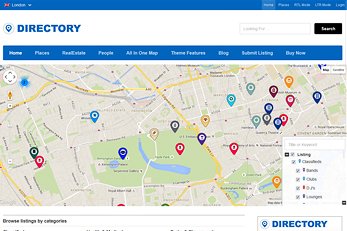A screenshot of a computer monitor showcases a cluttered and somewhat blurry directory interface. At the top of the screen, a blue navigation bar stretches across, fading into the distance. To the left, a conspicuous red icon with illegible white writing flanks the screen. The upper right corner displays a list of five words in white text, with only the word “log in” on the far right discernible.

Underneath this header, a white background highlights a teardrop-shaped blue pin next to a white circle. To their right, the word “directory” appears in dark blue lettering. On the far right, a search box is paired with a rectangular black search button.

A blue banner below showcases white labels, including “Home,” “Places,” “Theme,” “Features,” and “Buy More,” some of which are distinguishable through the blur. Beneath this banner lies a rectangular section depicting a Google map, peppered with multi-colored teardrop pins in red, green, gray, blue, and purple.

On the right-hand side, a white square acts as a legend for the map, filled with several words that are unreadable. Below this legend, a white bar reads “Browse listings by categories” in white text, accompanied by very small, blurry labels. In the bottom right corner, the word “directory” reappears in the same dark blue font.